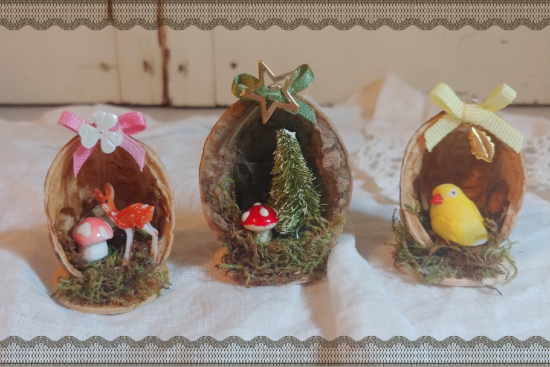The image showcases three decorative ornaments arranged on a white linen background with bluish-green rickrack on the edges. Each ornament, resembling a half egg or walnut shell, serves as a miniature diorama filled with enchanted forest scenes. 

- The left ornament features a light brown shell with a three-leaf white clover tied with a pink bow at the top. Within the shell, a deer figurine stands beside a red and white spotted toadstool, both nestled in a bed of moss.
- The middle, slightly larger, ornament displays a light brown shell adorned with a green bow and a gold-colored five-pointed star. It houses a small evergreen tree dusted with snow, accompanied by a red and white toadstool on a mossy base.
- The right ornament also has a light brown shell decorated with a yellow bow and a gold leaf. Inside, a small yellow bird with an orange beak, positioned to face the viewer, sits among moss and twigs. 

In the background, a white painted wall with a noticeable crack adds a touch of rustic charm, while additional rickrack borders the scene. Altogether, these ornaments create a whimsical depiction of a forest, captured with distinct detail and vibrant colors.